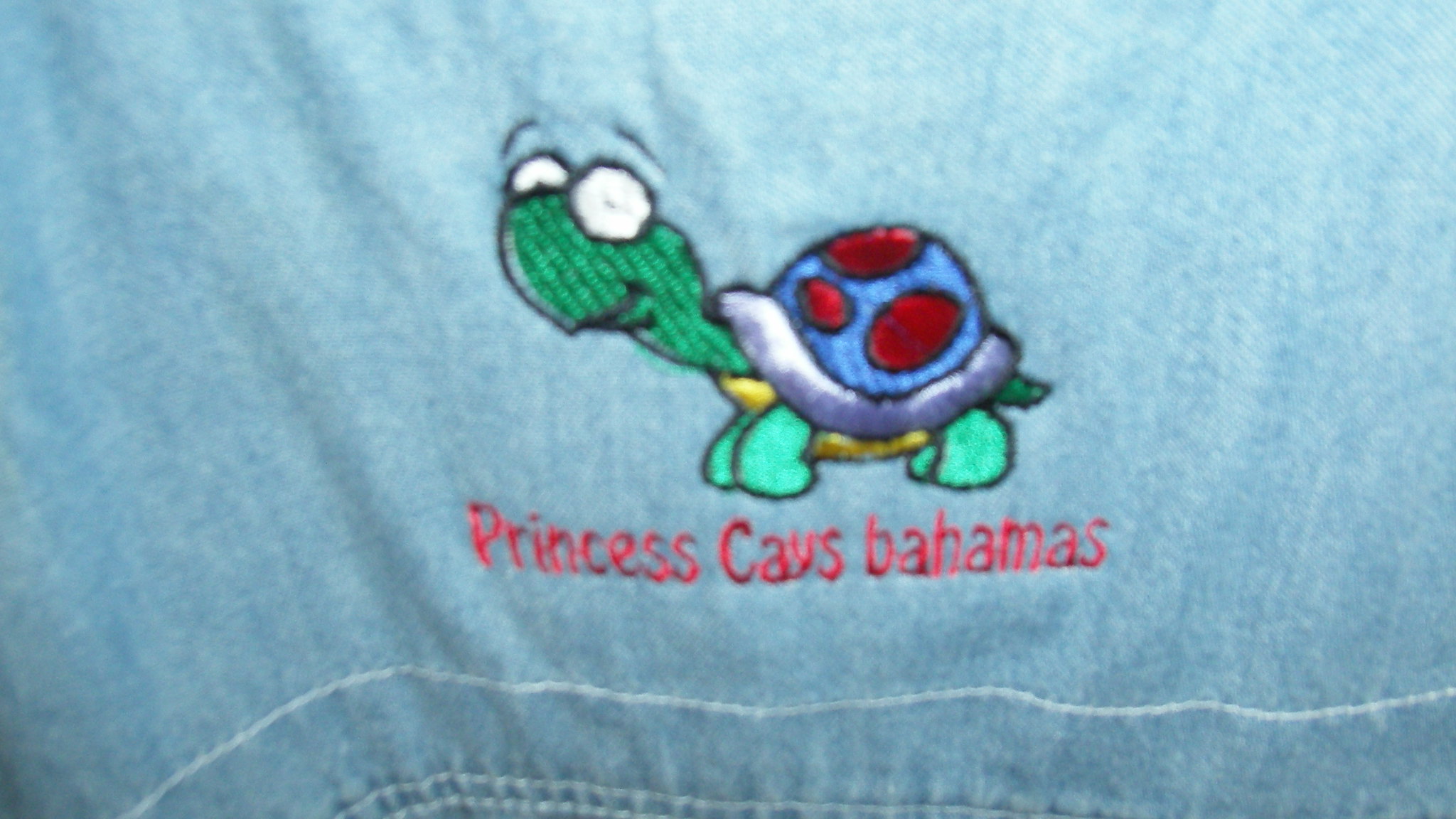This photograph showcases a finely embroidered design on a light blue denim fabric. At the bottom of the image, a small white seam adds a subtle touch to the overall aesthetic. The central feature is vibrant red embroidered text reading "Princess K's Bahamas." Above the text, there is a charming cartoon turtle, intricately detailed with a bold black outline. The turtle has a green head and legs, a yellow underbelly, and a distinctive shell edged in white. The main portion of the shell is blue, adorned with three striking red polka dots, adding a playful pop of color to the design. This delightful embroidery exudes a sense of whimsy and charm, perfectly capturing the essence of a tropical getaway.